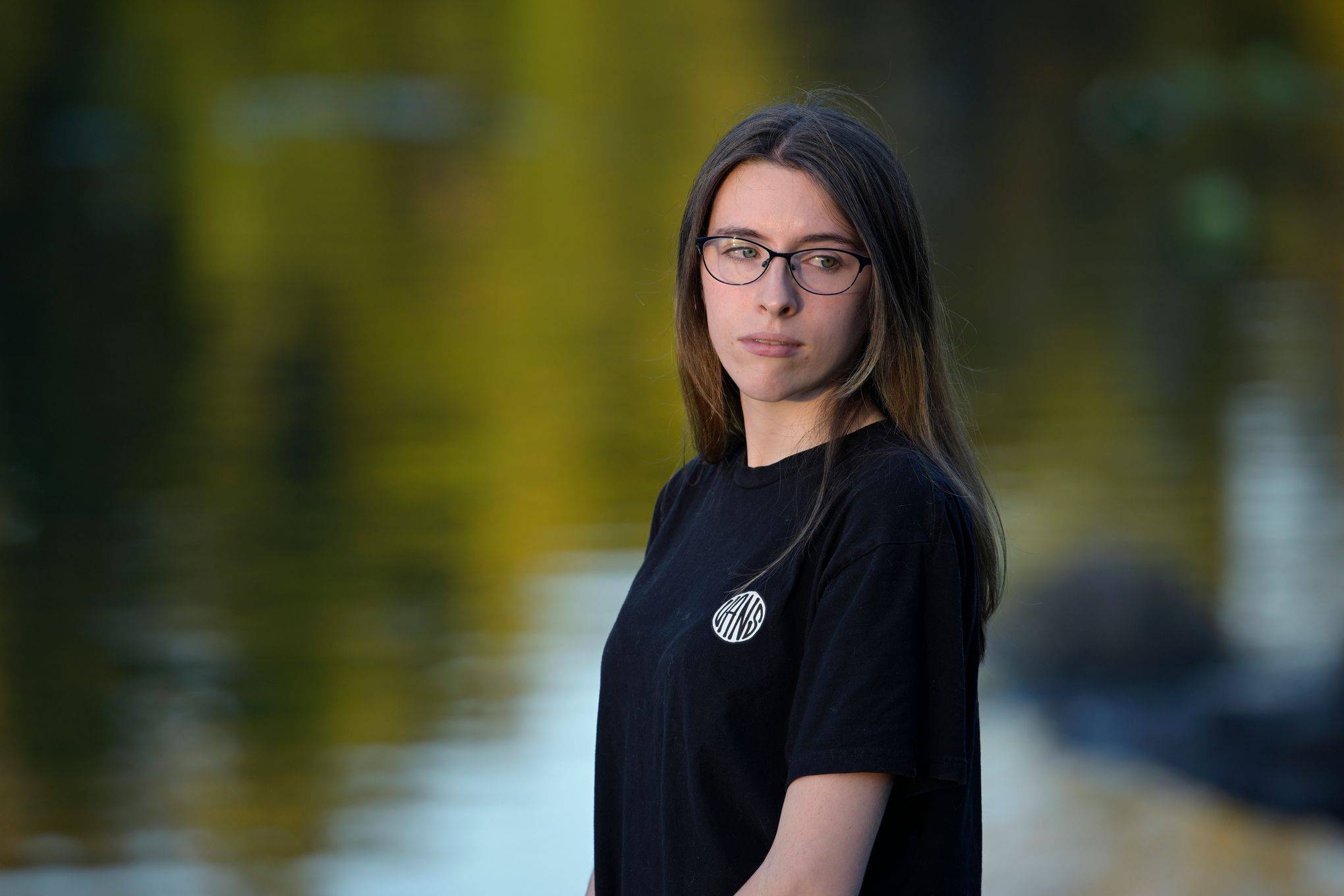This is a close-up photograph of a middle-aged Caucasian woman with fair skin and long, straight brown hair, which features subtle brown or slightly blonde highlights at the bottom. Her hair is parted in the middle and she is wearing black, round-rimmed glasses. She has a neutral expression and is gazing off to her right, seemingly at something in the distance. The woman is dressed in a short-sleeved black t-shirt with a small white circle logo featuring black text on the front right side of her chest, which appears to spell out "VANS." The background is blurred but suggests a reflective body of water, possibly a park lake with murky greenish-yellow hues. The reflections in the water indicate the presence of nearby trees.